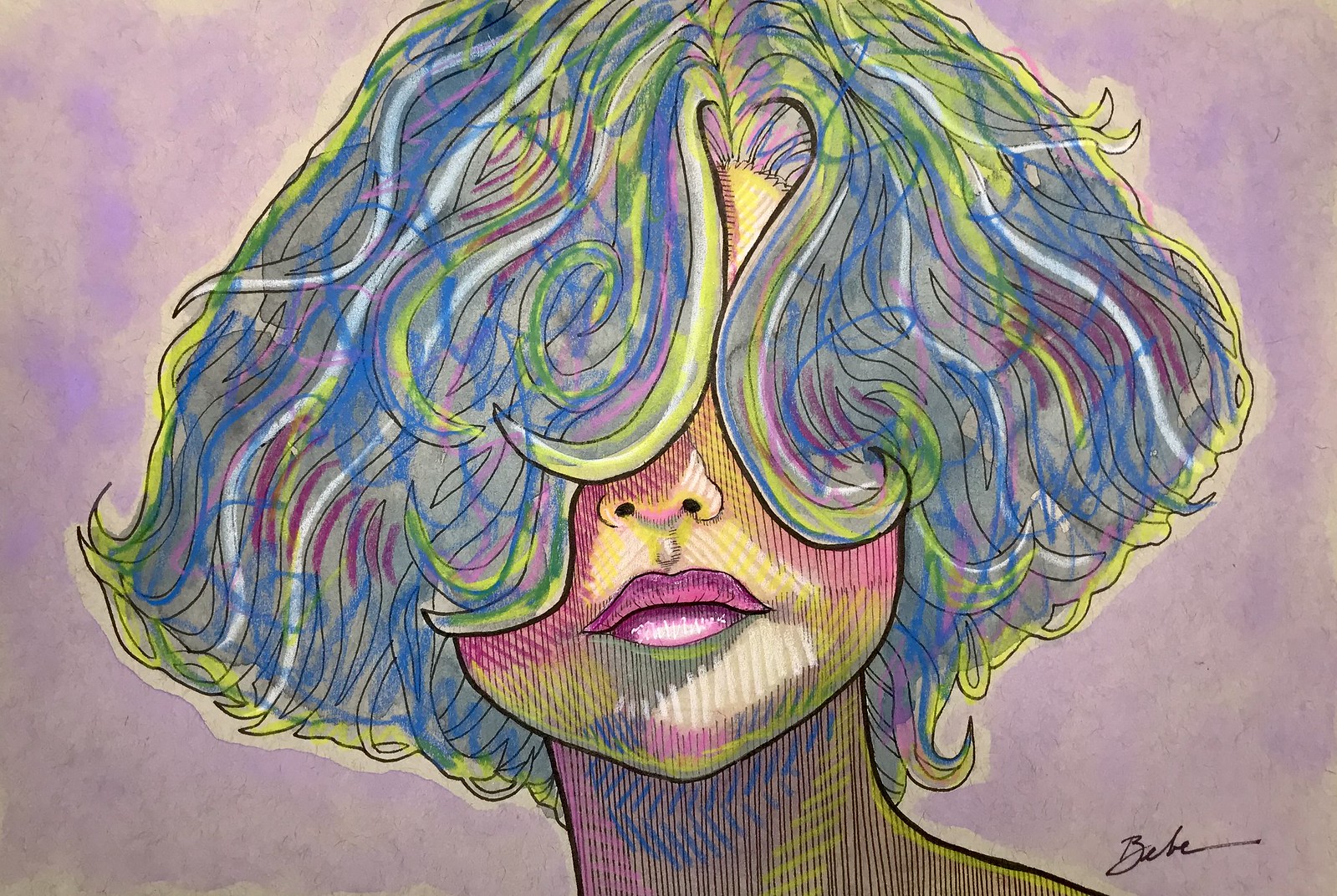The image is a digital artwork with a predominantly purplish background that features cloud-like imprints of lighter and darker shades. The main focus is the face of a woman with short, multicolored hair that descends in long bangs, obscuring her eyes and revealing only her nose, lips, and pointy chin. Her hair, chaotic and wavy, showcases a striking blend of colors including yellow, white, pink, red, blue, and green, outlined by a white haze. Her face carries multicolored shading, predominantly yellow with pink, red, green, and blue accents, including a large patch of white on her chin and light magenta lips. Her neck, covered in light blue chevrons and a mixture of blue, pink, and yellow shades, extends down to her shoulders. The bottom right of the image features a cursive signature that appears to spell "Bebe".